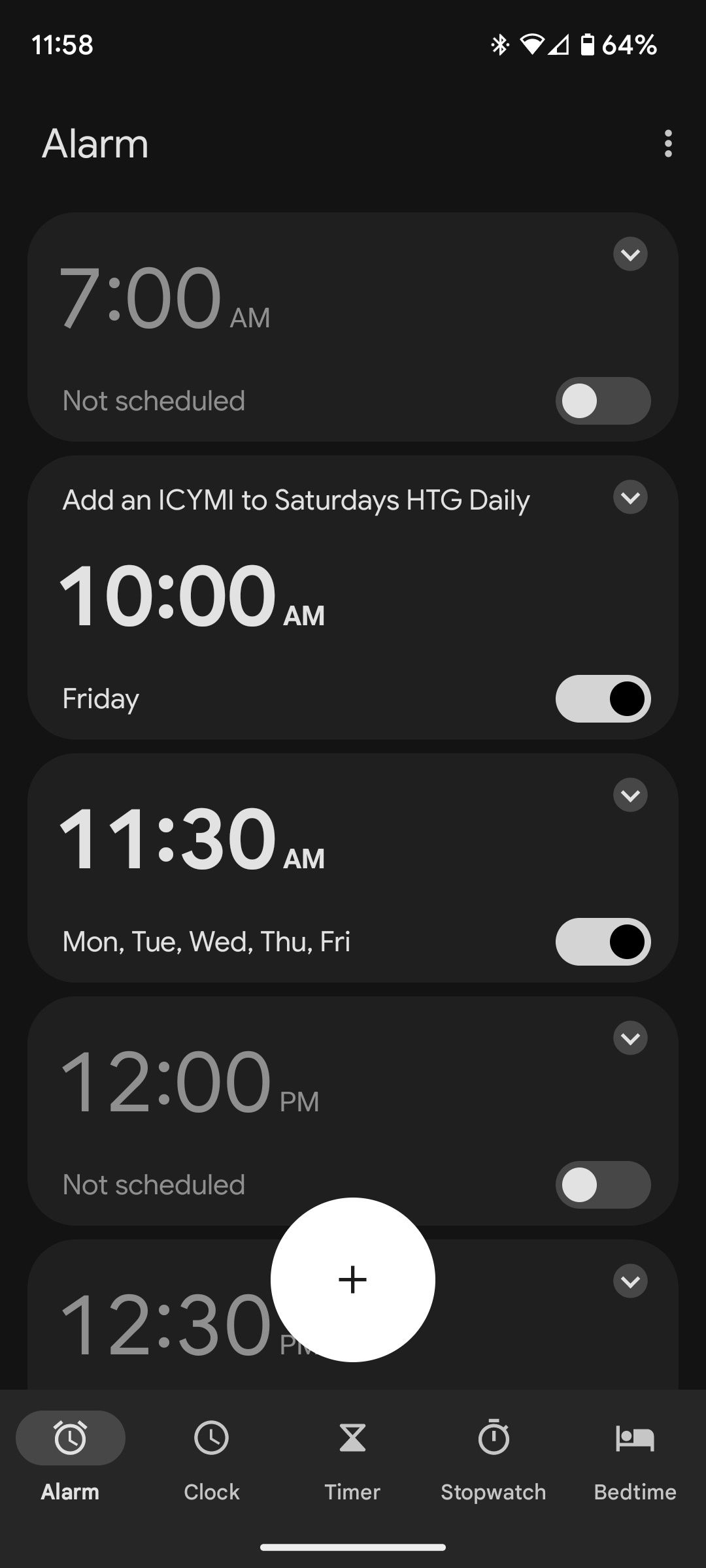The image displays a smartphone screen in portrait mode. The status bar at the top of the screen shows the current time, 11:58, in white text on the upper left. On the upper right, the Bluetooth icon, reception strength, Wi-Fi signal, and battery level indicators are visible, with the battery level at 64%.

The main content of the screen is a list of alarms. At the top left, the word "Alarm" is prominently displayed in white. Beneath this, five different alarms are listed:

1. The first alarm is set for **7:00 AM** but is marked as "Not scheduled" and the switch next to it is grey, indicating it is turned off.
2. The second alarm, written in white text, is labeled **"Add an ICYMI to Saturday's HTG Daily"** and is set for **10:00 AM Friday**. The switch next to it is white, indicating it is turned on.
3. The third alarm, also in white text, is set for **11:30 AM** on **Monday, Tuesday, Wednesday, Thursday, and Friday**, with the switch next to it white, showing it is activated.
4. The fourth alarm, for **12:00 PM**, is marked as "Not scheduled" and the switch is grey, indicating it is not active.
5. The fifth alarm is partially cut off but is for **12:30 PM**. Over this entry, there's a white circle icon.

At the bottom of the screen, navigation tabs labeled **Alarm, Clock, Timer, Stopwatch,** and **Bedtime** are visible, providing additional options for time-related functions.